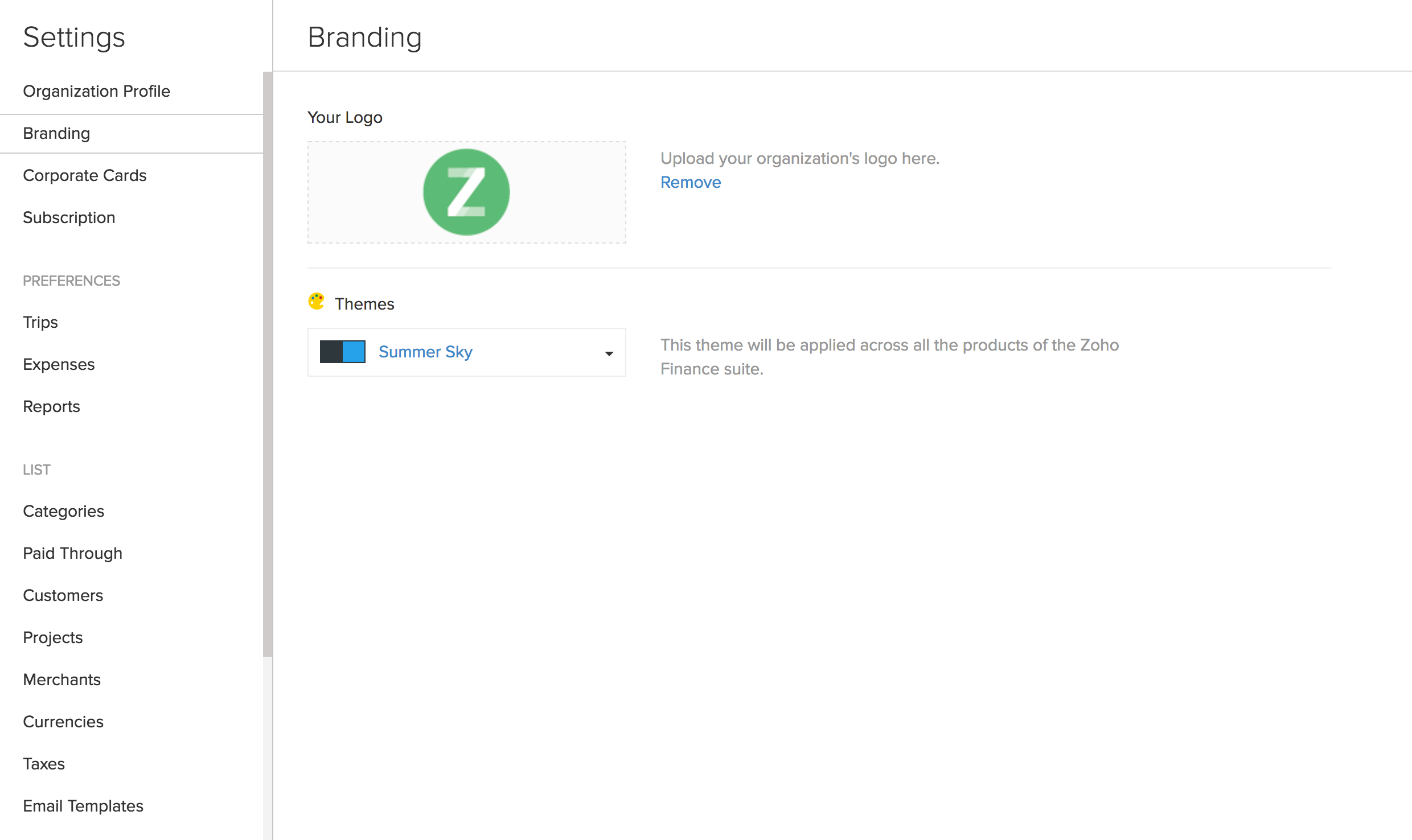The image is a screenshot captured from a desktop computer's screen displaying a white background interface with two window panes. On the left, a vertical navigation pane is titled "Settings" at the top and lists several options in descending order: Organization profile, Branding, Corporate cards, Subscription, Preferences, Trips, Expenses, Reports, Lists, Categories, Paid through, Customers, Projects, Merchants, Currencies, Taxes, and Email templates. The right section, which is larger, is the main content area. At the top of this pane, the word "Branding" is prominently displayed, followed by a faint grey dividing line. Below the line, the text "Your Logo" appears in smaller font size. Underneath "Your Logo," there is a small green circle housing a capital letter "Z."